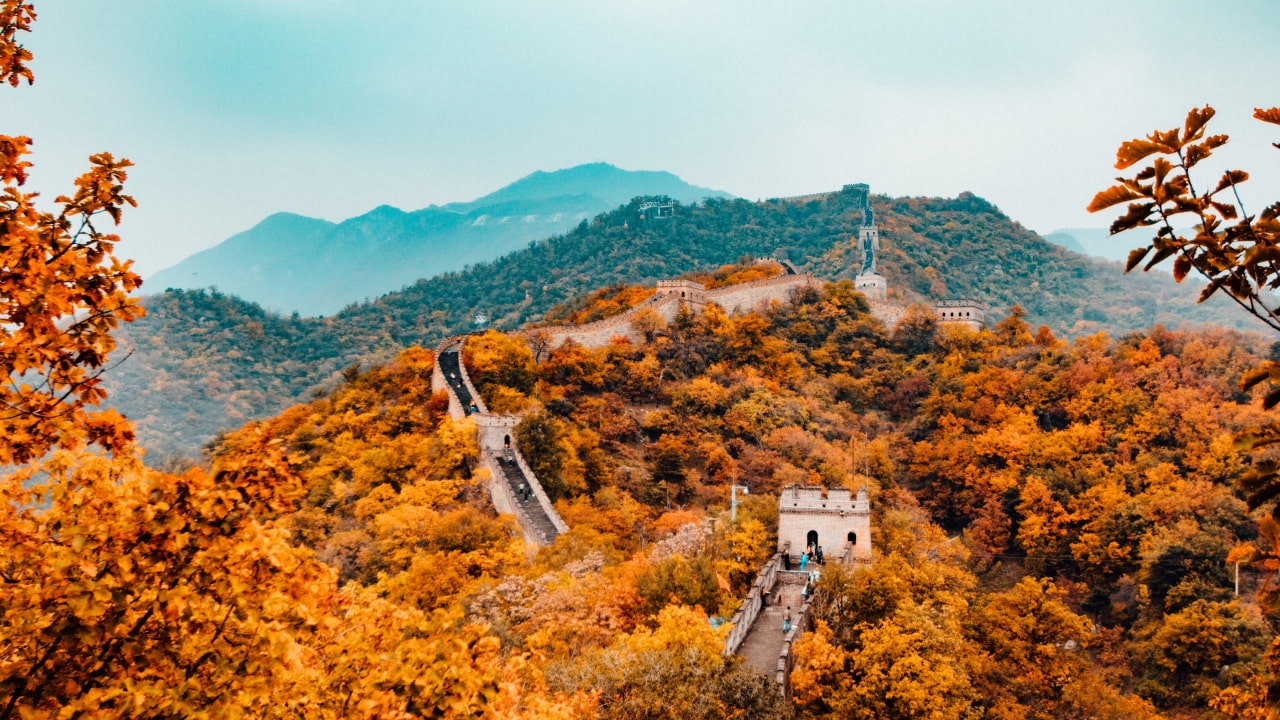This colored photograph vividly depicts the Great Wall of China amid a striking autumn landscape. The foreground is dominated by brilliant orange, yellow, and golden-hued trees, encapsulating the seasonal transition. The Wall itself snakes sinuously across rugged terrain, with its ancient battlements and watchtowers prominently visible. Pockets of people, some in blue shirts, are discernible on the Wall, albeit from a distance. As the Wall recedes into the background, it traverses through gradually darkening green foliage. The scene culminates in a misty, bluish-green horizon where mountains shrouded in fog blend with the grayish-blue sky, creating an ethereal atmosphere. This composition harmoniously frames the historical grandeur of the Great Wall against the vibrant and fading colors of the surrounding landscape, capturing a moment that is both timeless and transient.